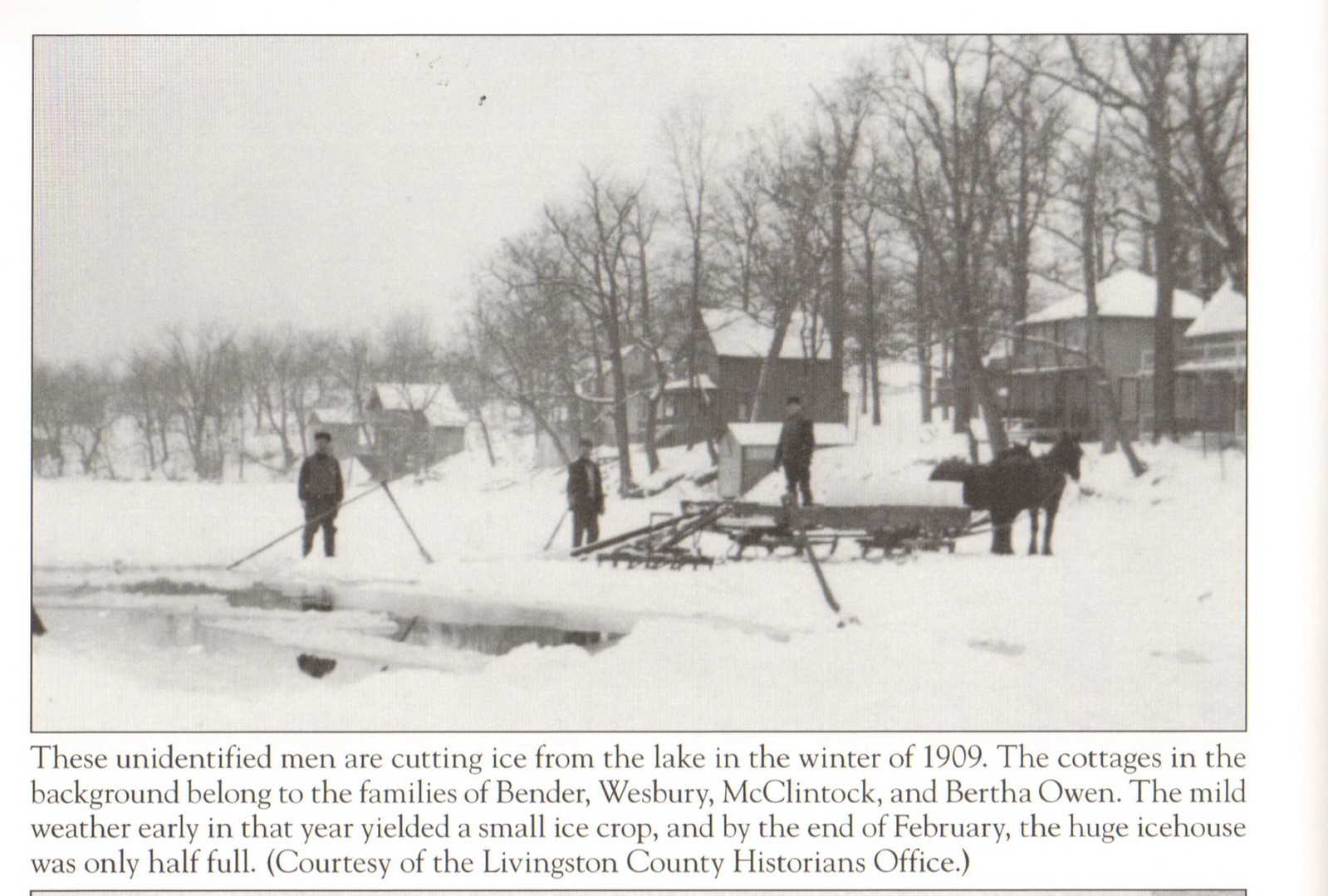The black and white photograph, dating back to the winter of 1909, captures a wintry scene of three men cutting ice from a lake. The setting is enveloped in snow, with the lake itself visible in the bottom left corner of the image. The men are positioned across the frame: one stands to the left near the lake, another stands to his right, and the third man stands on what appears to be a wooden sled designed for transporting ice. Attached to this sled are two horses, indicating their role in the ice-cutting process. In the background, the bare trees and several cottages—belonging to the families of Bender, Wesberry (or Westbury), McClintock, and Bertha Owen—are visible. Captions below the photograph provide historical context, noting that mild weather early in the year led to a smaller ice harvest, leaving the ice house only half full by the end of February. The image is archived with the courtesy of the Livingston County Historian's Office.